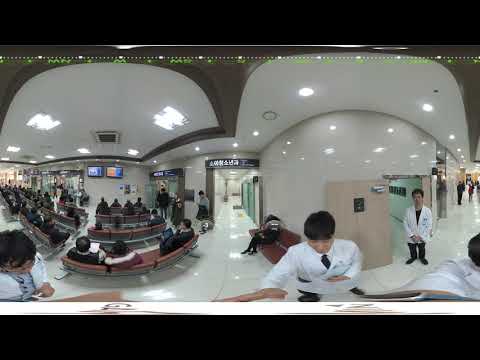The image depicts a busy hospital waiting area. The large room features four rows of chairs on the left side, most of which are occupied by people seated with their backs to the viewer. In front of these rows, there are two television monitors mounted on the wall, displaying content that is too blurry to identify. The scene extends into a long corridor, with a sign above written in an Asian language. The floors are white tile, and the walls are also white, complemented by recessed lighting in the ceiling. On the right side of the image, there are men in white jackets and black pants, possibly doctors or other medical professionals, as well as an open door propped open by a man who appears to be a staff member. The overall atmosphere is reminiscent of an airport departure gate, but distinctly medical, with a sense of organized activity and waiting.